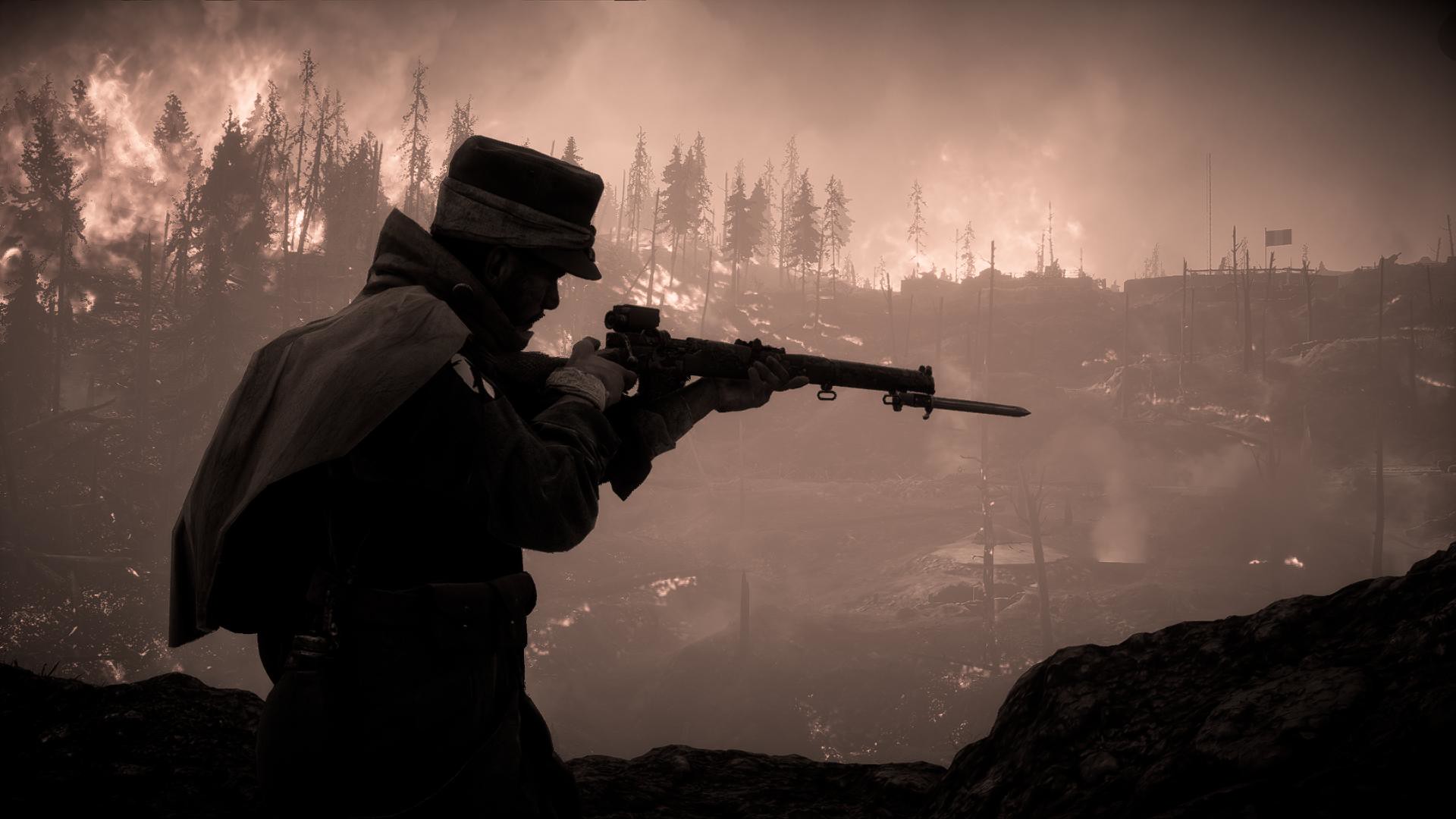This sepia-toned photograph depicts a wartime scene set outdoors, where chaos unfolds in both the foreground and the background. At the center, a soldier is prominently silhouetted in profile, aiming a rifle with a bayonet and a scope. He appears to be from a historical era, dressed in a coat and a hat adorned with a scarf. His gaze is intense as he points the gun upward, peering through the scope in a poised stance. He carries a backpack and firmly holds the rifle with both hands.

Behind the soldier, the sky is dark and tumultuous, with only a hint of light seeping through the dense layers of ominous black, dark gray, and light gray smoke. The background reveals a tall, thin tree line, possibly pine or evergreen trees, some of which are barren and burnt while others are engulfed in flames, indicative of a raging forest fire. The once lush greenery now sporadically covered with thin branches starkly contrasts with the fiery destruction.

At the lower part of the image, rocky outcroppings flank both corners, providing a rugged terrain that the soldier stands upon. A nearby building with a sign can be spotted amidst the rolling hill regions, some water bodies, and grassy patches interspersed with pools. This evocative scene merges the elements of nature and conflict, capturing a moment of historical warfare with striking detail.